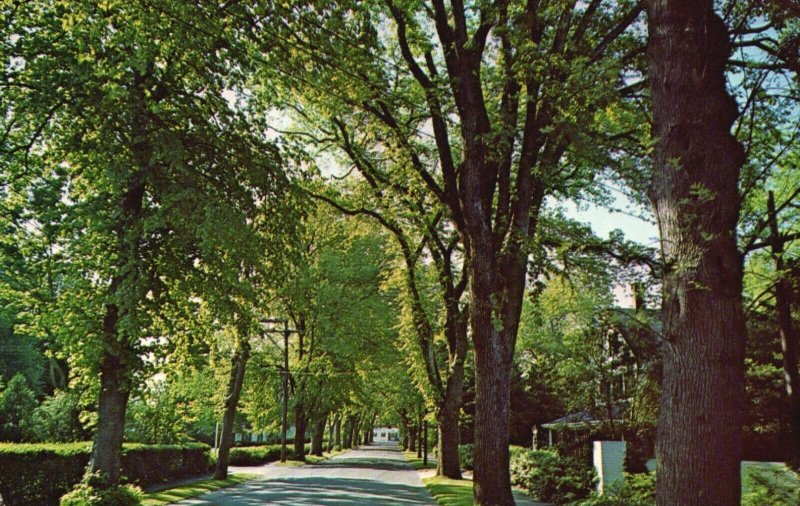The image depicts a serene, sunlit street scene, characterized by a wide, gray paved road with no cars or people present. Lining both sides of the street are tall, mature trees with thick trunks and lush green leaves that cast intricate shadows on the road. Blue sky with scattered white clouds frames the scene, adding to the tranquil atmosphere. On the right side in the background, there's a blue house with white accents, partially hidden by branches, accompanied by a gray porch roof. Further details include a white house somewhat concealed by branches and neatly maintained shrubbery along the sides. A brown telephone pole on the left with white wires stretching across the street adds to the array of elements. The main colors prominent in the image are black, white, blue, gray, brown, and various shades of green, contributing to a naturally picturesque and well-kept suburban landscape.